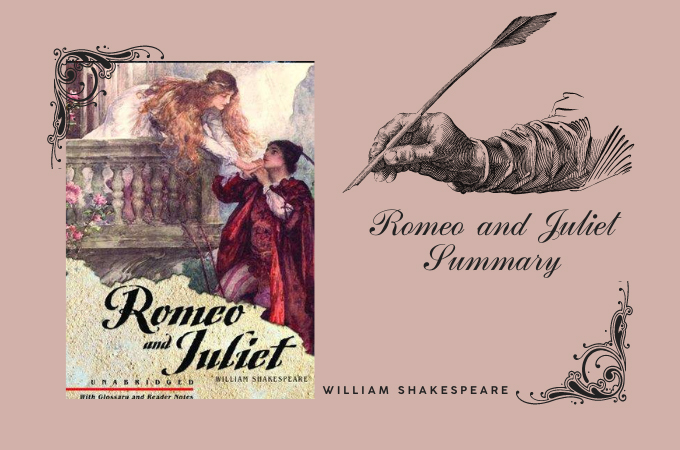The graphic, likely a slide from a presentation, features a rose-colored or pinkish pearl background. The left side displays a book cover of William Shakespeare's "Romeo and Juliet." The cover art depicts Juliet, dressed in a white gown with long blonde hair cascading over her shoulders, standing on a stone-walled balcony and leaning down to hold hands with Romeo, who is adorned in a red cloak, red shirt, purple, and white striped tights, and a black hat. He holds her hand from below, creating a romantic scene. The title "Romeo and Juliet" and "William Shakespeare" are prominently displayed at the bottom of this depiction.

On the right side of the slide, there's an ink pen illustration showcasing a hand holding a quill, detailed with a feather at the end. Below this drawing, in elegant cursive writing, it reads "Romeo and Juliet Summary." Additionally, the author's name, "William Shakespeare," appears at the bottom. Decorative graphics are situated in the corners, adding a touch of design to the slide which is presumably used in a classroom setting for summarizing Shakespeare's classic play.